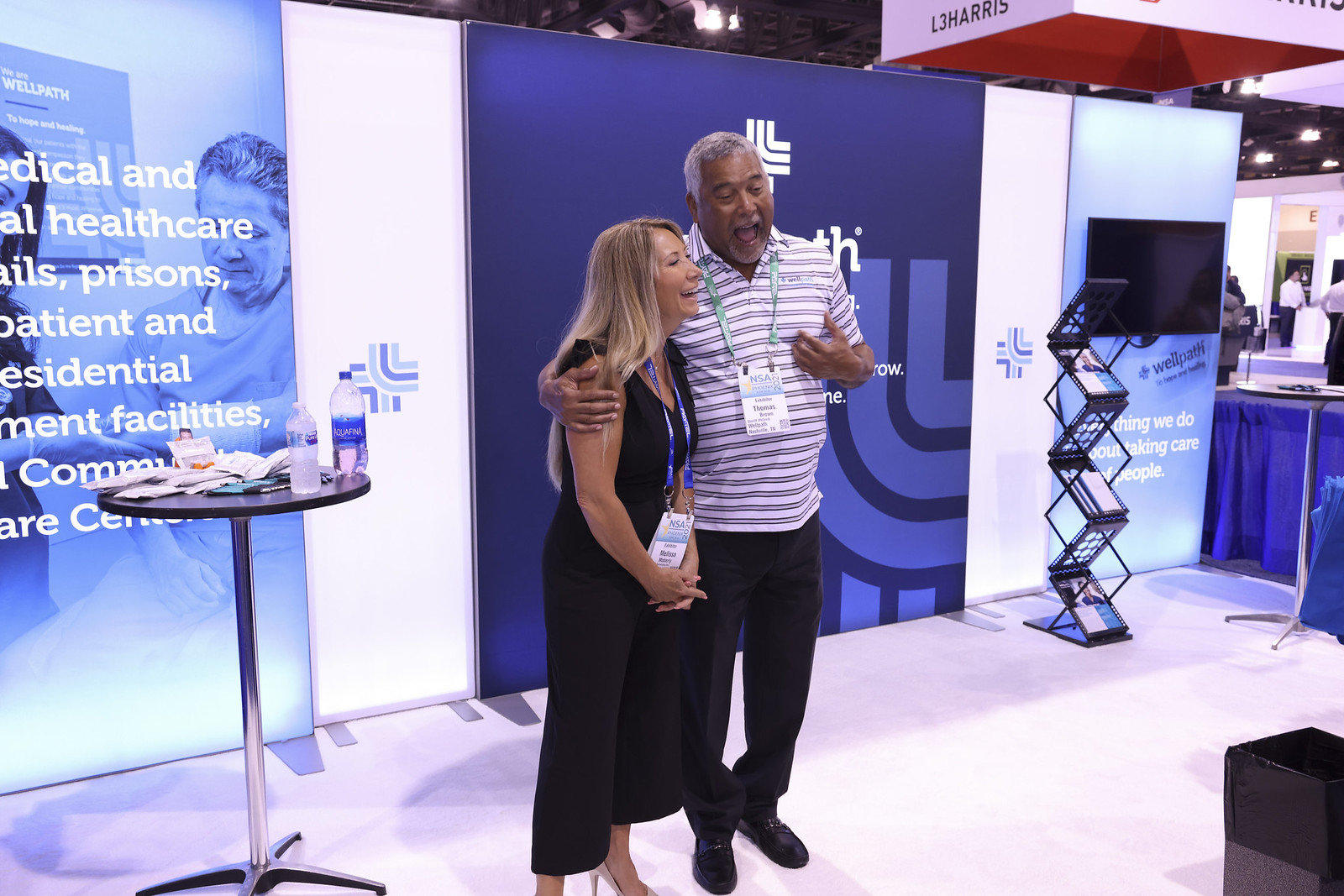In this wide rectangular image from a 2021 convention, two individuals, named Thomas and Melissa, stand on a white platform that starts at the bottom left and ascends diagonally to the right. Melissa, a white woman with long blonde hair, wears a sleeveless long black dress and grayish-mauve heels. Thomas, a Black man from Nashville, Tennessee, has his arm around her and is dressed in a white and black striped polo shirt over black pants and black shoes. Both have name tags, with Thomas's tag on a green lanyard and Melissa's on a blue one.

They appear to be laughing and making faces at someone off-screen, seemingly sharing a joke or a story. To their left is a round black table with two plastic water bottles, one labeled Aquafina, and several scattered plastic packets. Behind them is a wall adorned with various lit-up signs. One sign is dark blue with a white logo, and another features blue imagery with white text. There is also a TV screen with text partially visible behind the man, saying, "This thing we do about taking care of people."